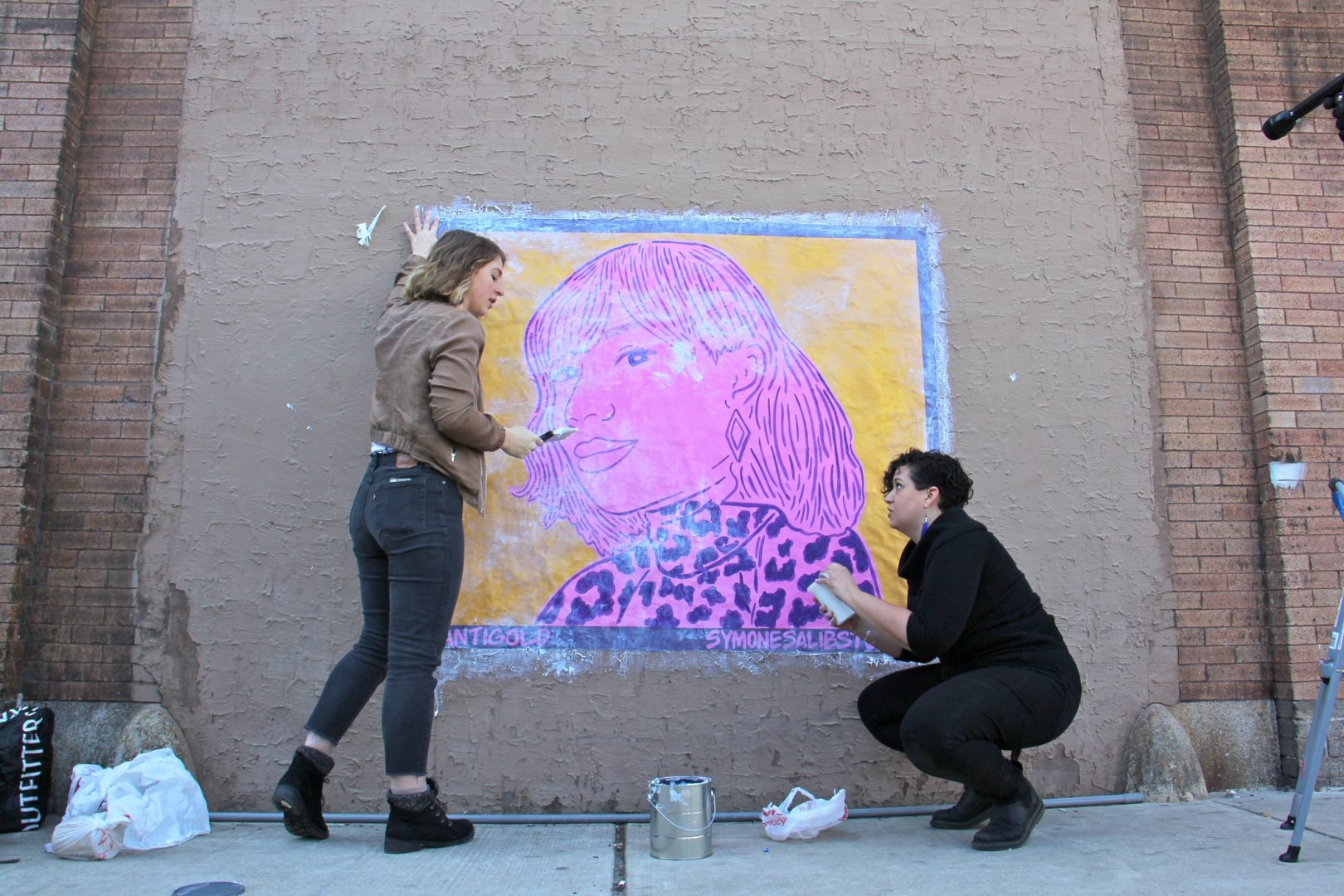The image captures two women engaged in painting a mural of Breonna Taylor on a brown brick wall that has been partially covered in a light tan stucco. The mural, which is centered, features a vibrant portrait outlined in blue, with a yellow background and hues of pink and black depicting Breonna Taylor. Taylor is illustrated with purple hair and wearing a leopard-patterned shirt. 

To the left of the mural stands a white woman with brown hair, dressed in blue jeans and a brown jacket, and holding a brush. She appears to be discussing the artwork with another woman on the right, who is dressed entirely in black with black boots, black jeans, and a black jacket, and is holding a cup or brush. At the bottom center of the image, a silver paint can sits between the two women.

Additional items include several bags on the bottom left and the legs of a mic stand with a microphone visible on the right side of the photo. In the background, part of the text on the wall reads "Antigold and Simone Salabast," though some of the text is obscured.